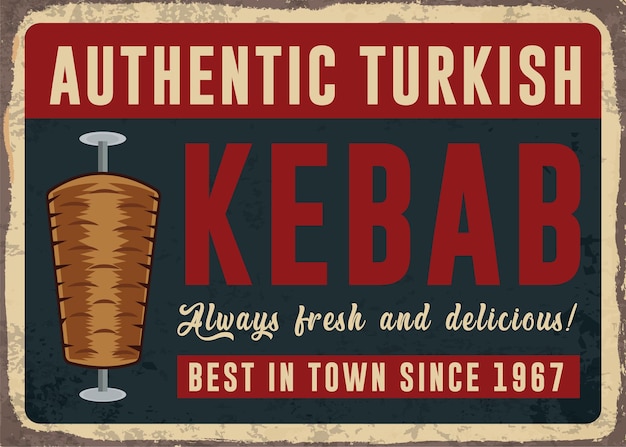The sign is a richly colored and vintage-style advertisement for a Turkish restaurant, featuring a detailed and eye-catching design. The overall shape is rectangular with dark brown edges and a weathered white border. At the top, the sign has a bold red section with white capital letters proclaiming "AUTHENTIC TURKISH." Directly beneath this, in a darker blue background, is the word "KEBAB" written in large, red, bold letters. Below "KEBAB", the sign continues with an inviting message in a stylish font: "Always Fresh and Delicious!" followed by "Best in Town since 1967" written in green. To the left of this text, there's a detailed illustration of a traditional Turkish kebab, resembling a cyclone-shaped piece of meat on a gray skewer, which adds an authentic touch to the advertisement. The overall color palette of the sign includes red, blue, white, cream, and brown, contributing to its retro and vibrant aesthetic.